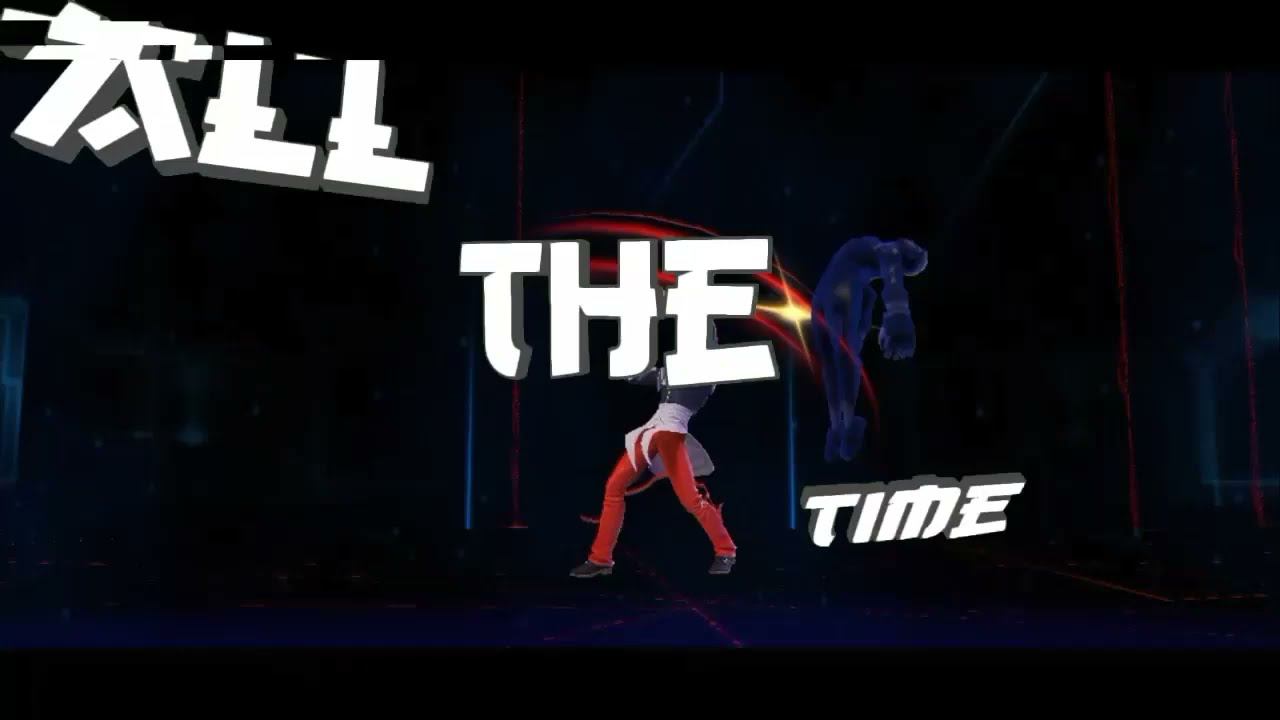The image is likely a screenshot from a futuristic fighting video game, showcasing a dramatic scene between two humanoid figures. The background is a dark blue and black gradient, setting a high-intensity mood. In the center, a character wearing red pants and a white and black coat bends backward, appearing to throw another figure over their head. This thrown figure is faintly outlined in indigo, with arms and legs flailing as though struck mid-air. Dynamic whoosh lines, accompanied by a yellow sparkle, arc over the head of the character in red, indicating motion. The scene is overlaid with large white, all-caps text in a samurai-style font: "ALL" in the top left, "THE" in the middle, and "TIME" in the lower right. Thin black borders enhance the dark, immersive atmosphere of the image.